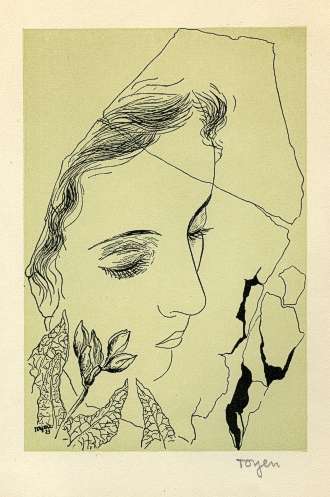This artwork is a detailed pen and ink illustration featuring the profile of a woman's face. Her eyes are closed, adorned with long black eyelashes and thin eyebrows, complementing her elegant features, which include a high nose bridge and defined lips. A portion of her wavy black hair is visible, with some of it hinted to be covered by an object or obscured. Beneath her face, a delicate arrangement of leaves frames a central flower. This flower is on the verge of blooming, with four unopened buds surrounded by three distinct leaves. The woman appears to be depicted within a coffin-shaped window, which has a crack along its right edge, and the background showcases an irregular, cracked paper effect accentuating the piece. The drawing is set against a light olive green backdrop, although hints of a yellowish hue and a pinkish-white border are also noted, possibly due to photographing or scanning artifacts. The artist’s signature, "TOYEN," is inscribed in handwriting below the lower right edge of the drawing, adding a personal touch to this meticulously crafted image.